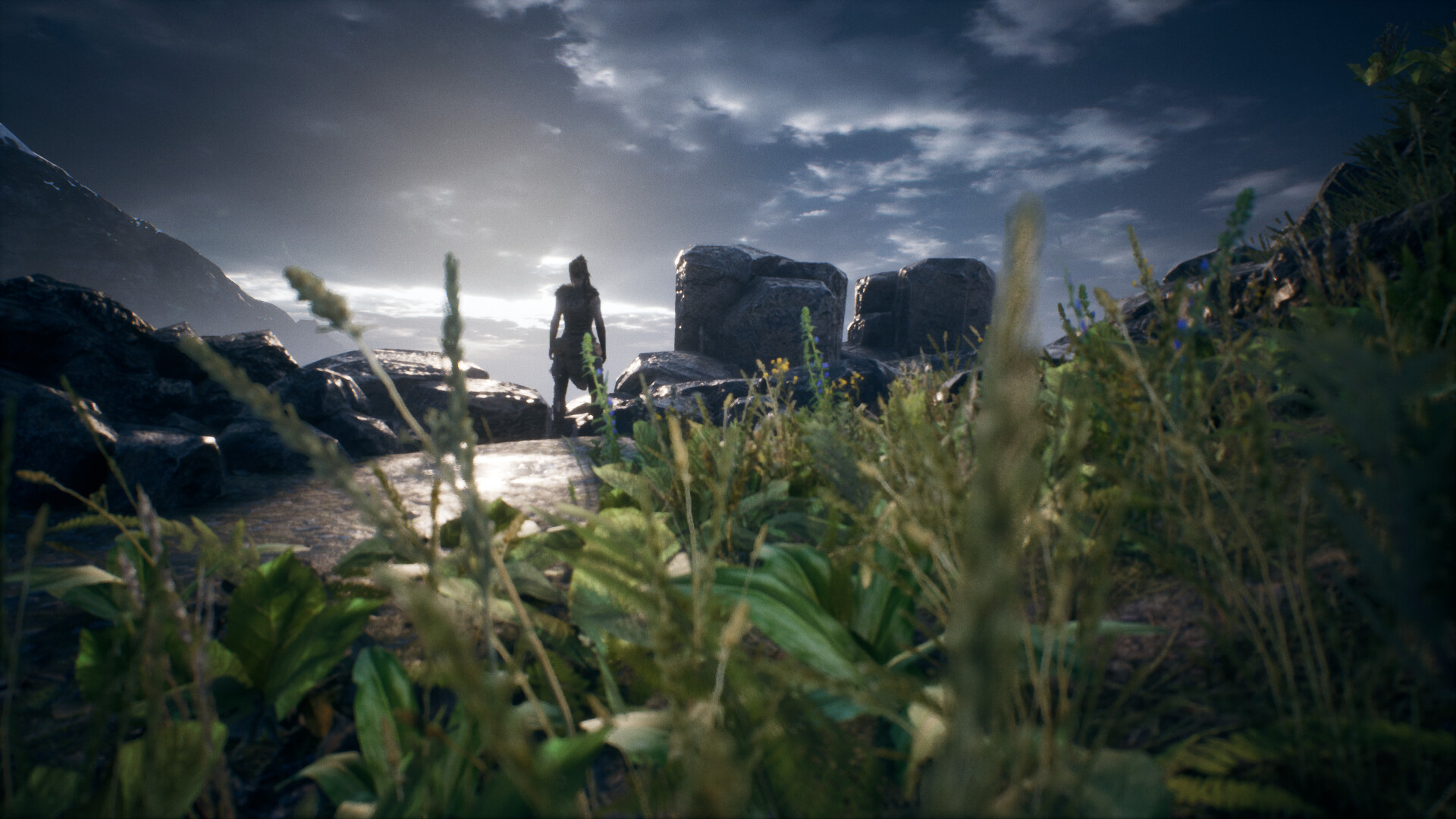This is an in-game screenshot from a video game that captures a highly immersive scene from a low, ground-level vantage point. The foreground features a patch of vibrant green grass, interspersed with tall, white stalks reminiscent of wheat. Scattered among the grass are several shiny, black rocks varying in size, some appearing almost life-sized. Next to one of the larger rocks, a shadowy figure of a woman can be seen, adorned in a distinct outfit that is difficult to detail due to the dim lighting around her. The background is dominated by a radiant sun, casting a bright light across the scene, and a sky filled with low-lying, ominous clouds in shades of black and white, adding a dramatic contrast to the entire composition.